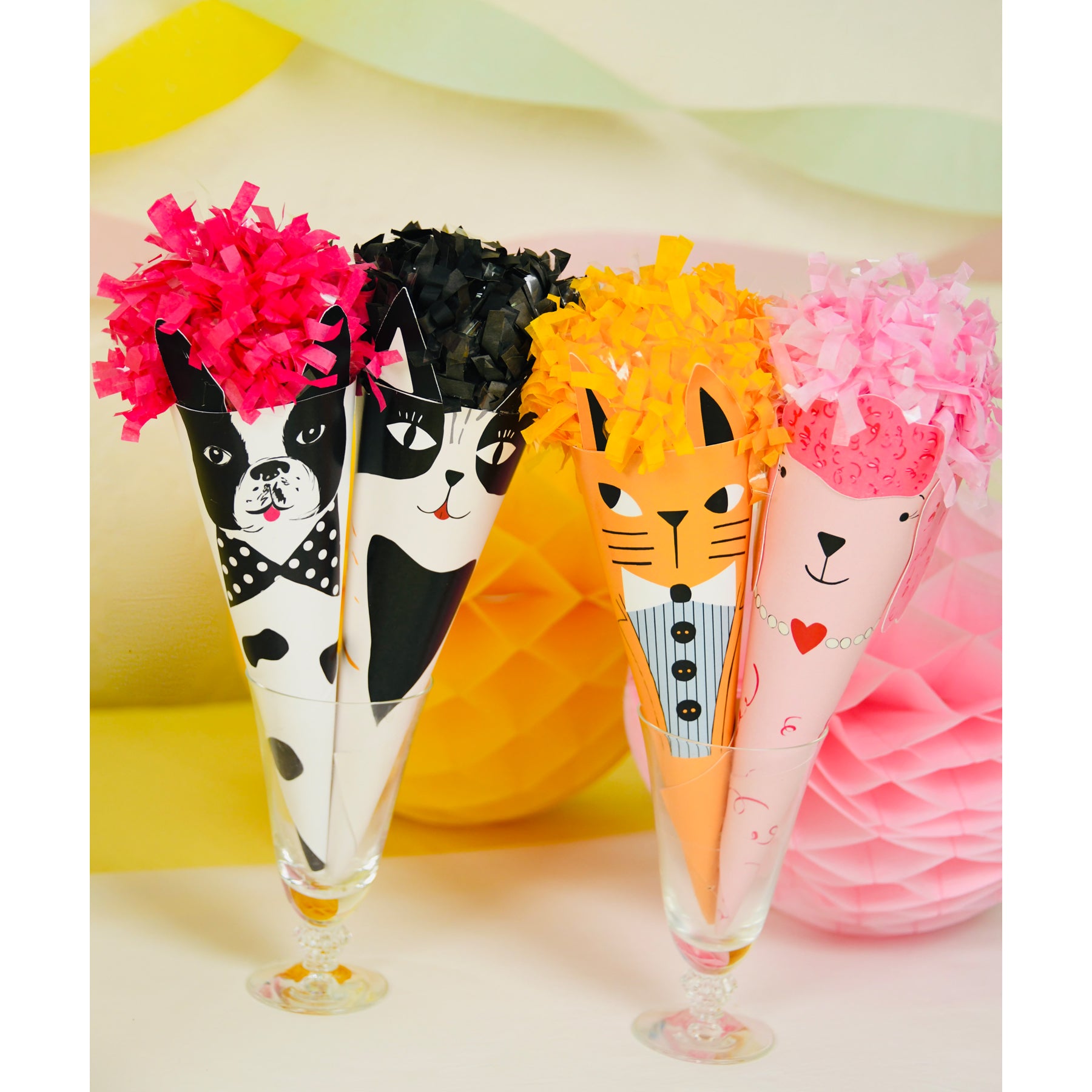This color photograph, in portrait orientation, features a close-up of whimsical party decorations arranged inside two conical-shaped glass goblets. These goblets are set prominently in the foreground, and each contains two paper conical noisemakers adorned with charming animal faces and topped with clusters of colorful shredded paper mimicking hair. 

In the goblet on the left, a black and white kitten with black accents under its chin and a contrasting black bulldog with pink hair are nestled together. The bulldog sports a black bow tie with white polka dots, while the kitten has striking facial markings.

The goblet on the right contains a vibrant scene with an orange cat donning an outfit styled with a blue and white striped shirt and collar, looking to the left. Accompanying it is a playful pink poodle, distinguished by its red heart pearl necklace and joyous smile, crowned with matching pink shredded paper hair.

In the background, decorative paper art balls in orange and pink hues add to the festive atmosphere, subtly hinting at the folded, spherical designs that contribute to the overall celebratory mood of the image. This photograph exemplifies photographic representational realism, capturing the intricate details and textures vividly.